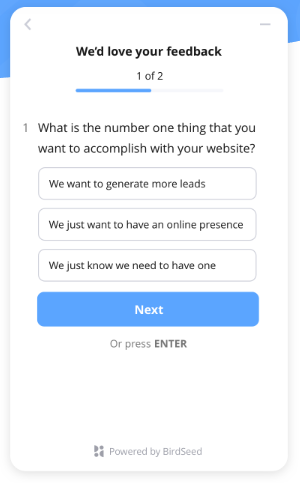A mobile screenshot showing a customer feedback survey from a company or app, designed to gather user input. The interface features a predominantly white background, punctuated by a light blue accent at the top, and side margins, which are a little more prominent on the left. In the top left corner, there's a light gray arrow pointing to the left, suggesting a return or back function.

Centered prominently below the arrow in bold black text is the phrase, "We'd love your feedback." Directly underneath, it indicates "1 of 2," implying it is the first of two questions in the survey. The first question asks, "What is the number one thing that you want to accomplish with your website?" 

Three clickable options are provided in bubble format:
1. "We want to generate more leads,"
2. "We want to have an online presence," and
3. "We just know we need to have one."

A noticeable blue button with white text invites users to proceed to the next page. Below this button, additional navigation instruction reads, "or press enter." At the very bottom, the survey is branded with the text, "Powered by Birdseed."